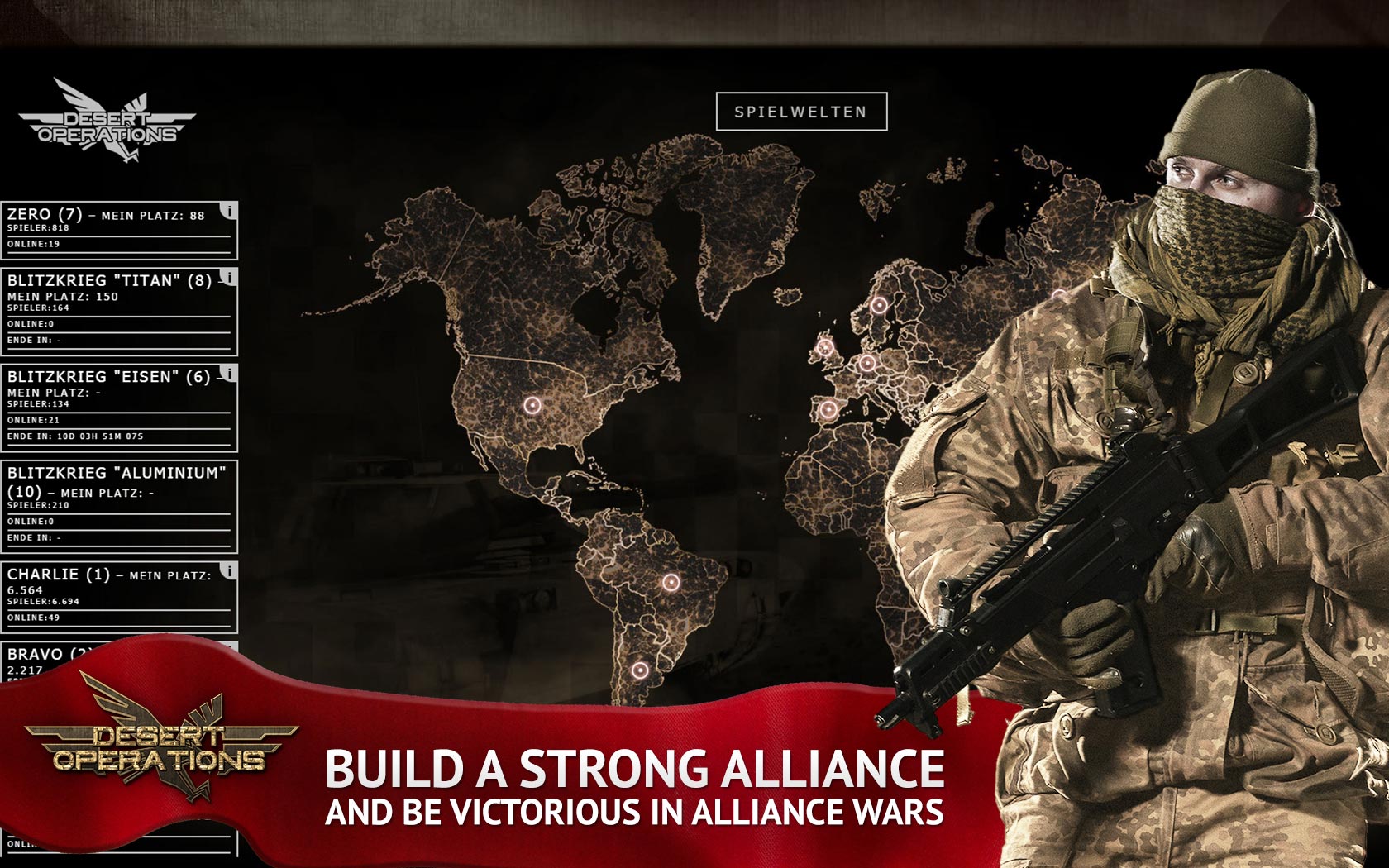The image is a horizontal advertisement for the military strategy game "Desert Operations." Prominently featured on the right side is a soldier dressed in a brown and dark green camouflage uniform, complete with a green beanie and a scarf covering his face up to the nose. He is holding an all-black rifle and stands against a backdrop of a world map colored in black and brown. The map appears annotated with various texts related to missions, such as "07," "Charlie 1," and "Bravo."

In the upper left corner, the "Desert Operations" logo is displayed, featuring a flying eagle clutching guns. This logo is repeated in the lower left corner on a red background with bold, white uppercase letters. Beside this logo at the bottom, text reads: "Build a strong alliance and be victorious in alliance wars." The color scheme of the image incorporates shades of red, white, black, dark green, gray, and brown, creating a cohesive military aesthetic. Overall, the advertisement communicates the game's emphasis on strategy, alliances, and military engagement.